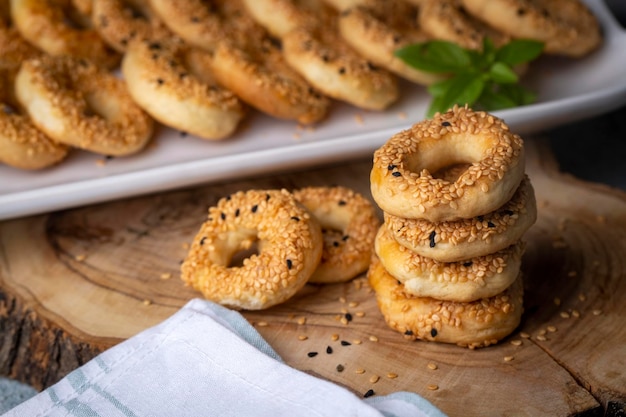In the photograph, a collection of mini bagels, adorned with a mix of sesame and a few stray black sesame seeds, are displayed on a rustic wooden log slice that serves as a natural table. The bagels exhibit a slight yellow tint, suggesting a perfect bake. On the log slice, four bagels are stacked neatly, while another set of two bagels are piled on top of each other. Various sesame seeds are scattered around the wooden surface. Adjacent to the stack, a white kitchen towel with green stripes is visible in the bottom left corner. Beside this arrangement, more bagels lean against each other on a large white porcelain platter, which is garnished with a green leaf. The scene, rich with texture, showcases these inviting and ready-to-eat baked delights.